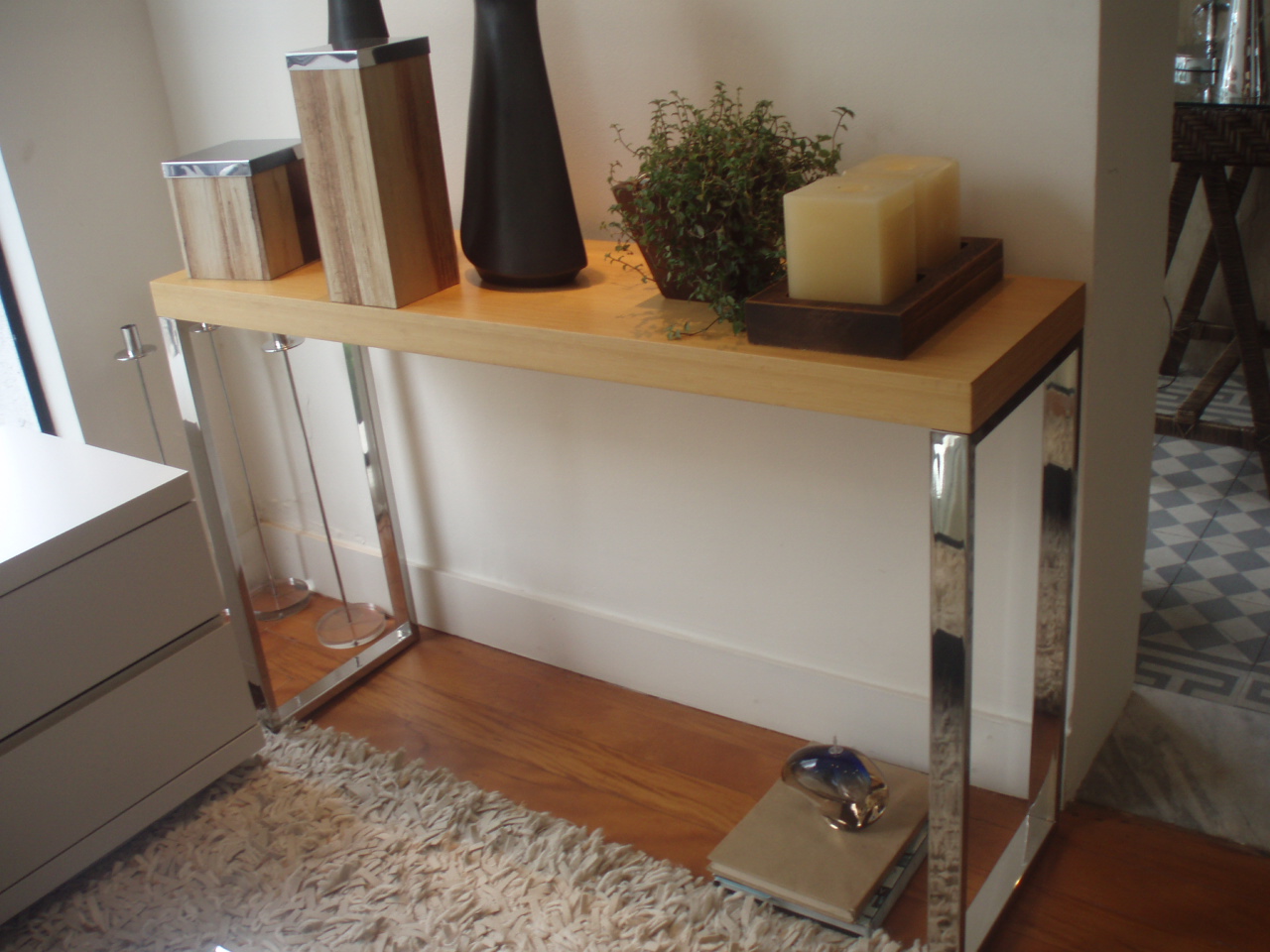The image showcases an interior home setting featuring a long accent table with a wooden top and shiny chrome legs. Positioned prominently, the table is adorned with modern decorations including two square ivory candles in a wooden tray, a small plant in a basket, and two dark vases. Additional items on the table include two decorative boxes with silver lids that resemble tree trunks. Below the table, resting on a wooden floor, there are three metal candle stands holding clear glass vases, along with two books and a clear glass decorative piece. Adjacent to the table is a white nightstand with drawers, and a cream-colored shag rug adds texture to the floor. The scene extends into another room past the white walls, presenting a harmonious blend of modern decor and natural elements.